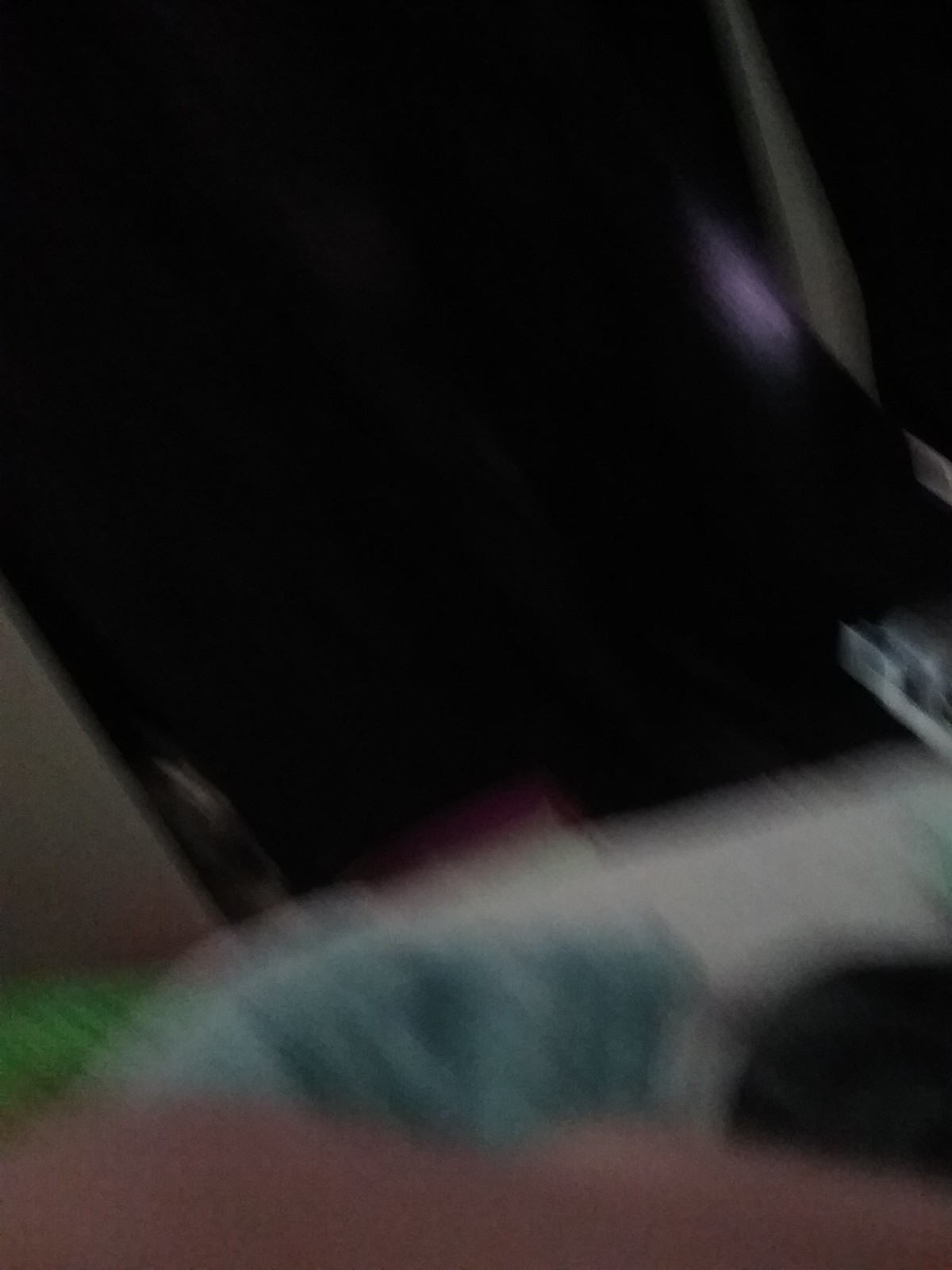This is a very blurry and dark photo with indistinguishable shapes and colors. Centered along the bottom is a dark flesh-colored bump, likely a hand, spanning across the entire corner. Above it, there's a patchwork of various colors: prominent areas of blue, green, red, and white stretching horizontally from left to right. To the left of this colorful band, there's a distinctive brown triangle shape. The majority of the image is enveloped in black, particularly covering the bottom left and the central upper left, which continues diagonally towards the bottom right. In the top right corner, there are noticeable streaks of purple and a larger light grayish mark. A black circle is present in the bottom right corner, situated between the flesh-colored strip and the white patch. Overall, this image appears to be a result of an accidental motion blur, rendering any specific subject or scene completely unrecognizable.